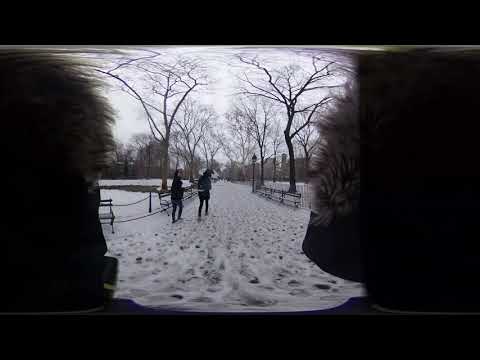The photograph captures a snowy city park with a long, snow-covered path lined with benches and lampposts on either side. The sky is overcast, casting a gray hue over the scene. In the center of the image, two people in winter clothing are walking away from the camera, making their way down the path; one appears to glance back towards the lens. Both individuals are blurred, adding to the serene yet mysterious atmosphere. The park is mostly devoid of other visible people, though there may be a distant, indistinct group at the far end of the path. The ground and path show numerous footprints, indicating that others have traversed this route despite the cold. Scattered dead trees stand starkly against the white landscape, enhancing the wintry feel. The image's color palette is predominantly white, black, and varying shades of gray, with perhaps a hint of brown, reflecting the somber, wintry setting in daylight.